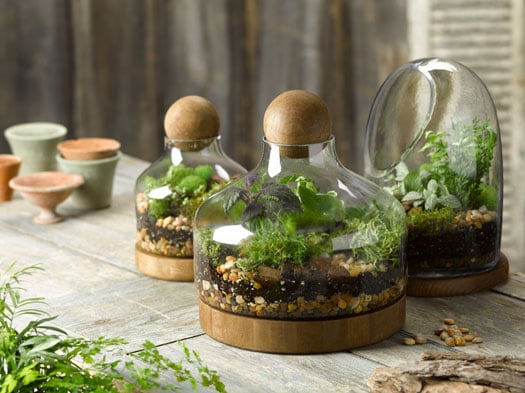This indoor photograph showcases three intricately crafted terrariums placed on a wooden table. Two of the terrariums are nearly identical, with rounded glass bodies tapering to a narrow top, sealed with a wooden ball, reminiscent of old-fashioned wine jugs. Both contain layers starting with pebbles at the base, followed by nutrient-rich soil, and topped with a mix of tiny green and red plants varying in leaf size. The third terrarium, positioned to the right, features a dome shape with a large cutout, housing the same pebbles, soil, and plant mixture. Surrounding the terrariums are small empty clay pots, some stones, and additional plants that extend onto the table, creating an impression of a miniature indoor garden workspace.